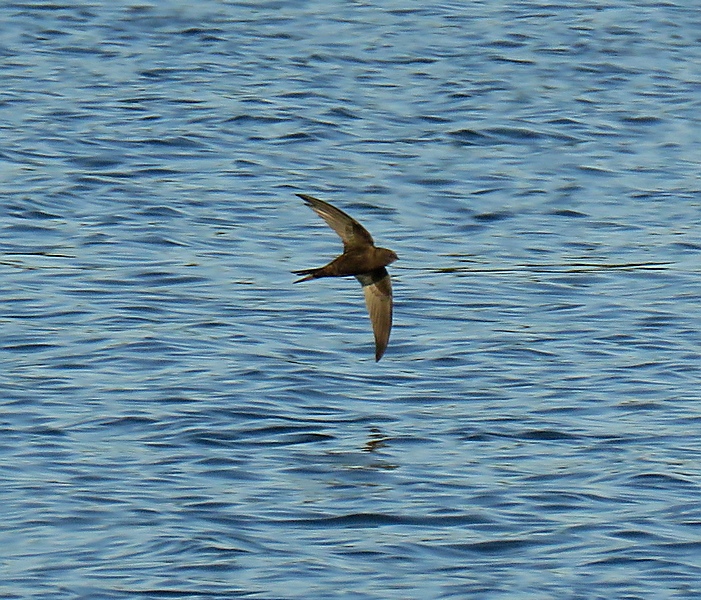In this detailed image, we see a serene yet subtly undulating body of water, likely either a lake or the ocean, as it stretches across the entire frame with varying shades of blue punctuated by dark blue flecks and small ripples. Dominating the center of the image is a small swallow, captured mid-flight as it glides swiftly from the left to the right. The swallow's brown body is contrasted by its distinctive V-shaped tail spread out behind it, and its small, dark eye and black bill are clearly visible. The bird's wings are fully extended, with the top wing swept back. The top wing transitions from white near the edges to a darker hue closer to the body, and the bottom wing dips towards the water, showing a gradient from whitish highlights in the sun to a dark gray-black shade nearer the water. The swallow's dynamic presence and extended wingspan cast a reflection on the water below, adding delicate black streaks to the subtly shifting palette of the waves.